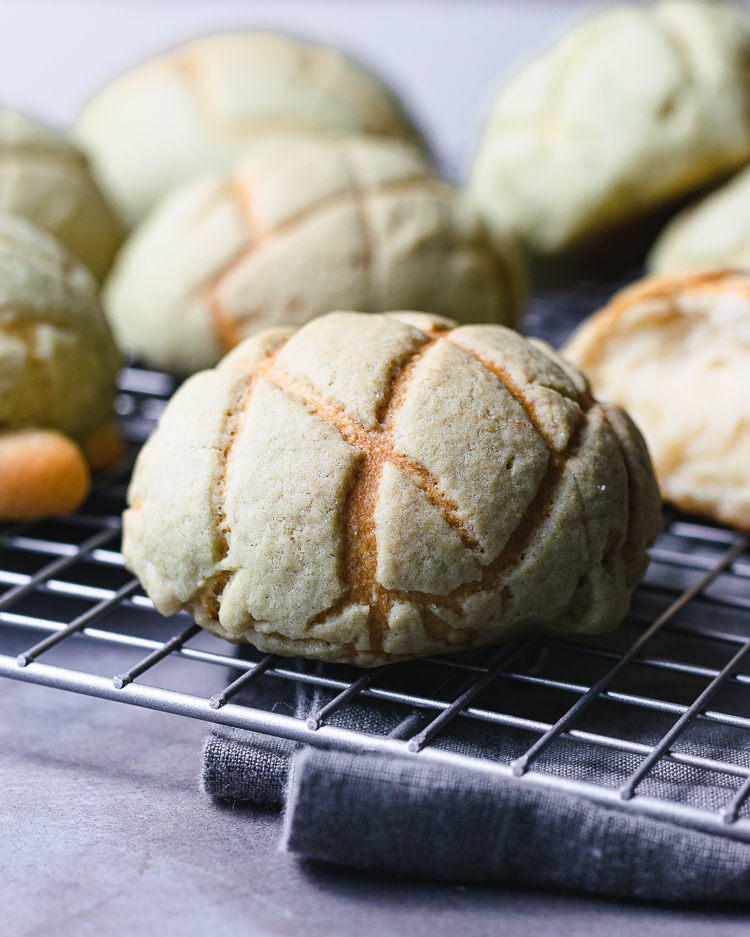This image showcases a collection of freshly baked Mexican pastries, likely conchas, arranged on a silver cooling rack. The pastries, characterized by their light beige color and distinctive dark brown scored lines, are set crisply in the foreground while the background blurs out. Center stage is a round, tan pastry with a brain-like appearance, complete with defined dark brown lines. Nearby, a similar pastry reveals its interior, having been broken open. Two additional pastries, slightly obscured and darker in color, appear to the left, while more conchas are scattered in the background. The silver rack rests on a folded blue towel, which in turn sits on a light gray table. The composition, accentuated by professional lighting and a soft focus effect, emphasizes the detailed textures and artistry of the pastries.